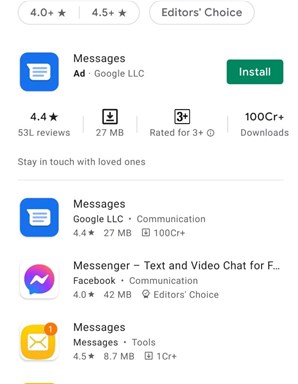The image displays a screenshot of a Google App Store interface, set against a white background and captured within a small rectangular frame. At the top of the webpage, star rating filters are visible, starting with "4.0+" on the left, followed by "4.5+" stars, and then "Editor's Choice" in black text. 

Just below these filters, a prominent app titled "Messages" is spotlighted. To its right is a green rectangular button labeled "Install." Beneath the "Messages" app logo, there is a 4.4-star rating accompanied by "53L reviews" and a download size specified as "27 MB." The app's brief description, "stay in touch with loved ones," is displayed right below this information.

Further down, three additional square-shaped app logos appear in succession. The sequence includes "Messages" again, followed by "Messenger" and "Facebook Messenger," and then another instance of "Messages." The second "Messages" app, appearing in blue, is noted as developed by "Google LLC." The last "Messages" app features a yellow logo with a white letter or envelope inside the yellow square, with just “Messages” written underneath, and no further details.

The space surrounding the apps and logos is characterized by a clean, pure white background, emphasizing the apps' visual presentation.